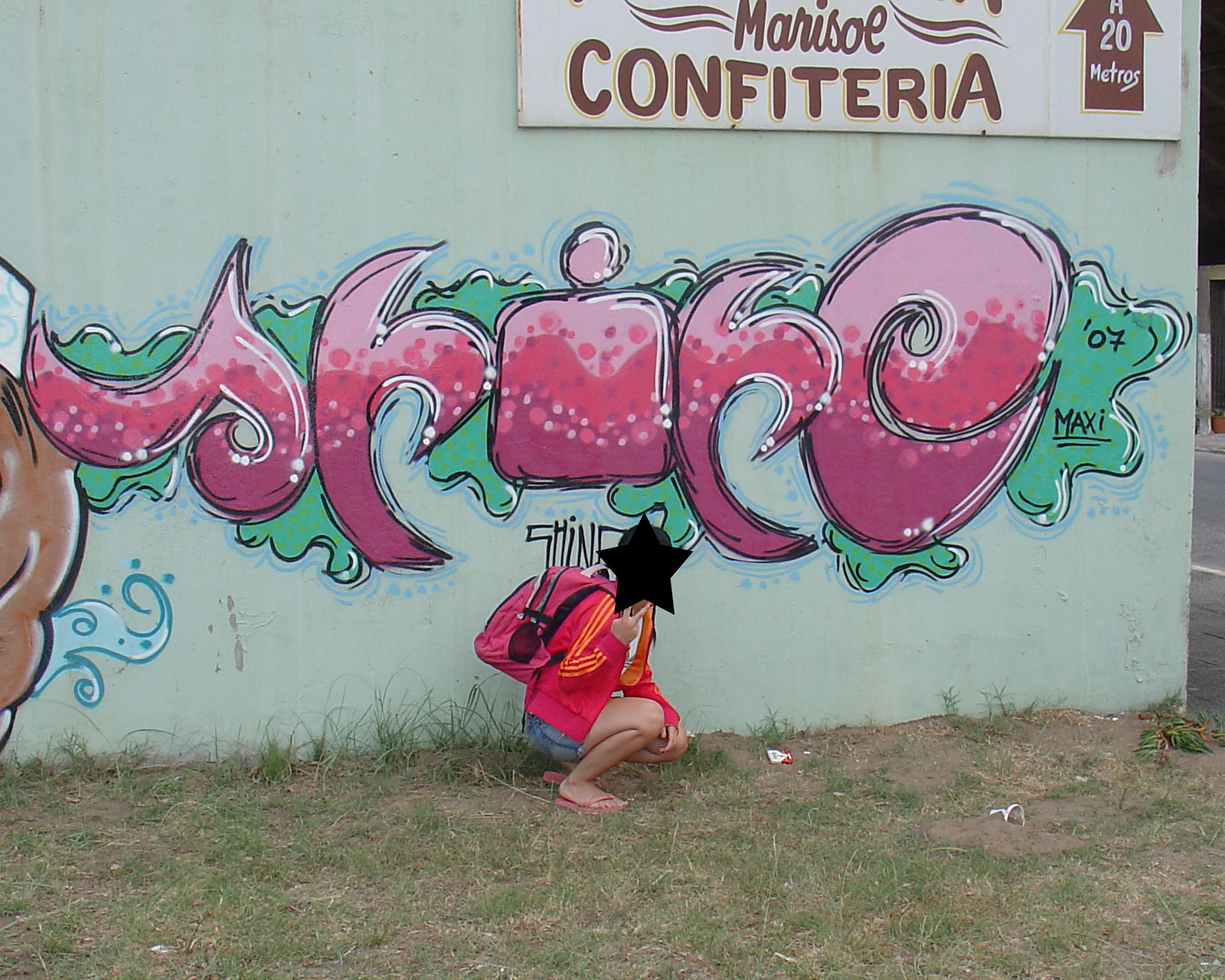The photograph depicts the side of a mint-green building adorned with vibrant graffiti. The graffiti, characterized by bubble-style letters, features a complex blend of pink, purple, magenta, and darker pink hues with green accents as the background. The letters, although hard to decipher, appear to spell out something like "SRIICE" or "YHICE," and include the tag "07 Maxi." Above the graffiti, a sign reads "Marisol Confiteria, 20 metros," with an arrow indicating direction.

In the foreground, a person squats on a grassy strip in front of the wall. The individual is dressed in a pink and orange jacket with yellow stripes on the sleeves, pink flip-flops, and jean cut-off shorts. They carry a pink backpack, and their face is obscured by a black star, which adds an element of anonymity. A road is visible to the right side of the image, enhancing the urban setting of the scene.